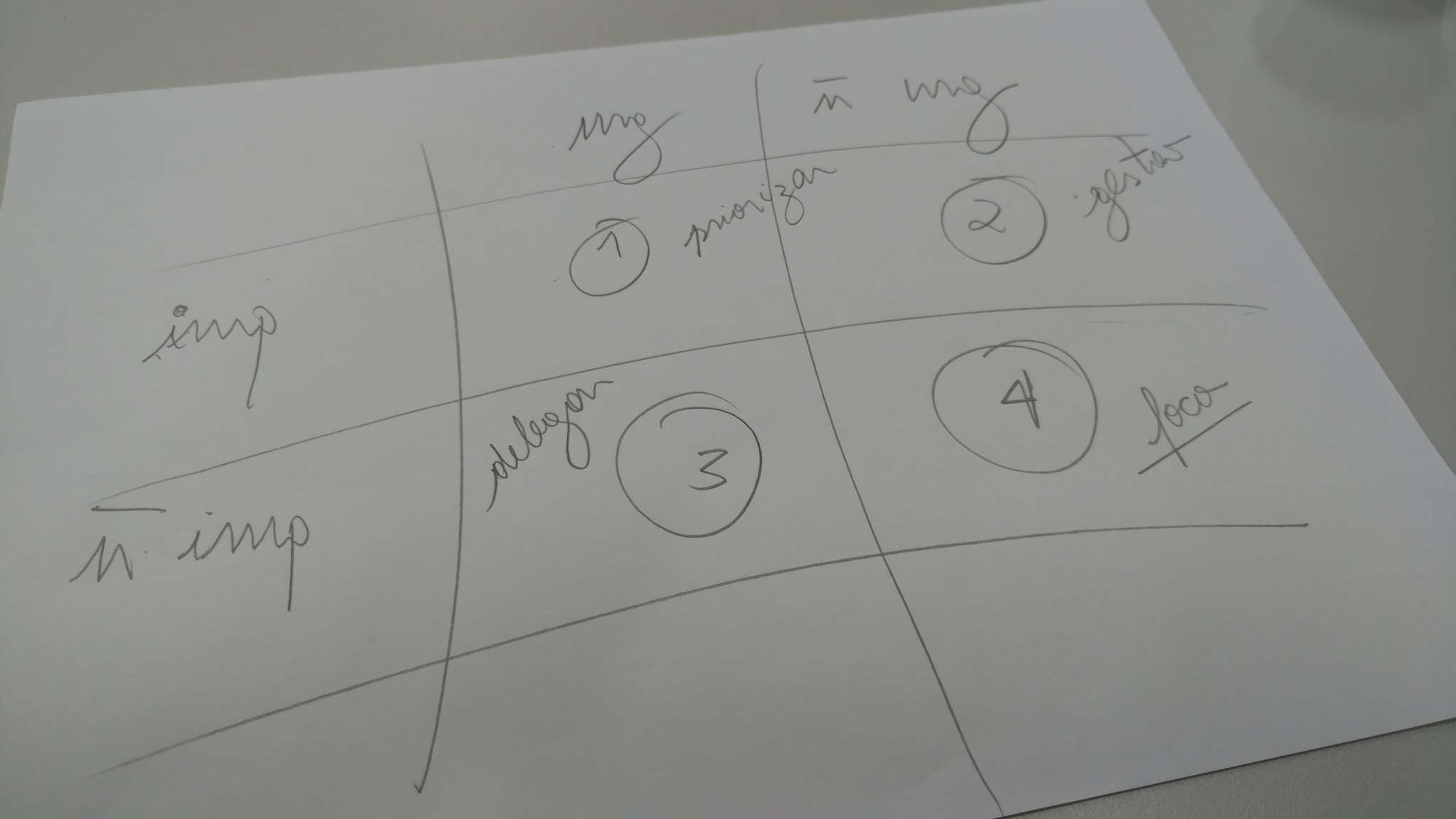The image features a piece of paper with a hand-drawn table consisting of three horizontal lines and two vertical lines, forming a grid structure. The table appears to be intended for organizational purposes. The handwriting on the page is in cursive, making some of the text difficult to decipher, but the words "imp" and "mimp" are clearly visible. The handwriting is legible but not particularly neat. Within the table are four distinct boxes, labeled and circled with numbers 1 through 4. Box 1 is located in the second row, second column; Box 2 is positioned in the second row, third column; Box 3 is in the third row, second column; and Box 4 can be found in the third row, third column.